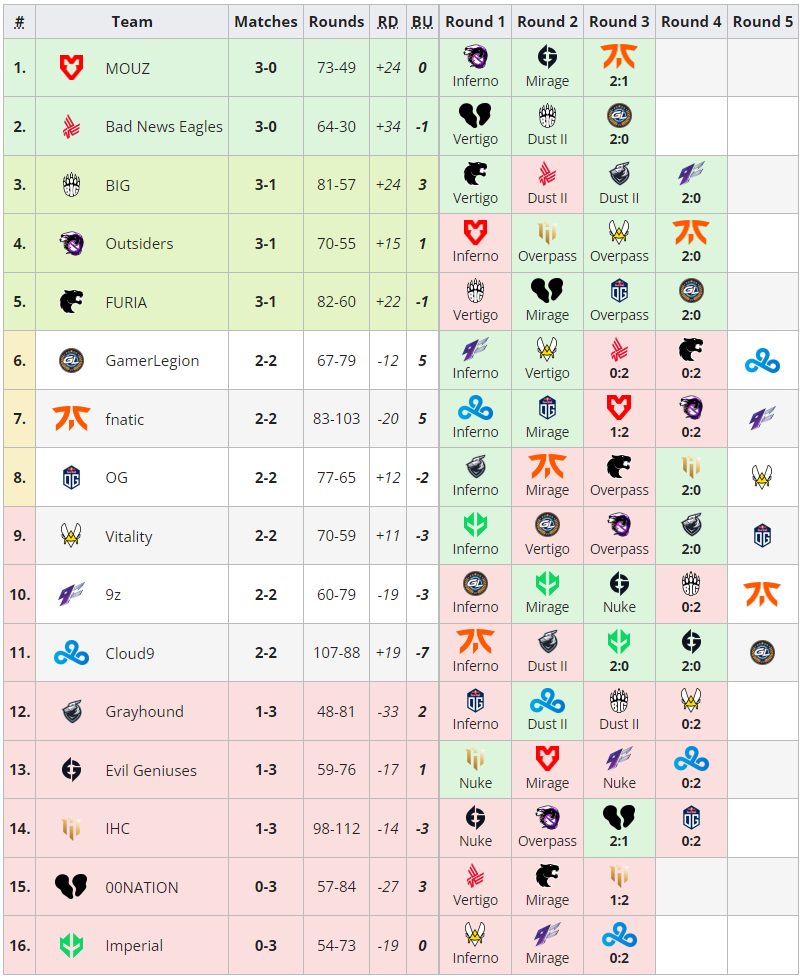**Detailed Tournament Standings Overview**

This detailed screenshot showcases the standings of teams from an unspecified tournament, highlighting various statistics across multiple columns: Team, Matches, Rounds, RD (Round Difference), BU (unknown), Round 1 to Round 5.

1. **MOUZ:** 
   - Matches: 3-0
   - Rounds: 73-49 
   - RD: +24
   - BU: 0
   - Rounds Breakdown: Inferno, Mirage (2-1)

2. **Bad News Eagles:**
   - Matches: 3-0
   - Rounds: 64-30
   - RD: +34
   - BU: -1
   - Rounds Breakdown: Vertigo, Dust 2 (2-0)

3. **BIG:**
   - Matches: 3-1
   - Rounds: 81-57
   - RD: +24
   - BU: 3
   - Rounds Breakdown: Vertigo, Dust 2, Dust 2 (2-0)

4. **Outsiders:**
   - Matches: 3-1
   - Rounds: 70-55
   - RD: +15
   - BU: 1
   - Rounds Breakdown: Inferno, Overpass, Overpass (2-0)

5. **FURIA:**
   - Matches: 3-1
   - Rounds: 82-60
   - RD: +22
   - BU: -1
   - Rounds Breakdown: Vertigo, Mirage, Overpass (2-0)

6. **GamerLegion:**
   - Matches: 2-2
   - Rounds: 67-79
   - RD: -12
   - BU: 5
   - Rounds Breakdown: Inferno, Vertigo (0-2, 0-2)

7. **Fnatic:**
   - Matches: 2-2
   - Rounds: 83-103
   - RD: -20
   - BU: 5
   - Rounds Breakdown: Inferno, Mirage (1-2, 0-2)

8. **OG:**
   - Matches: 2-2
   - Rounds: 77-65
   - RD: +12
   - BU: -2
   - Rounds Breakdown: Inferno, Mirage, Overpass (2-0)

9. **Vitality:**
   - Matches: 2-2
   - Rounds: 70-59
   - RD: +11
   - BU: -3
   - Rounds Breakdown: Inferno, Vertigo, Overpass (2-0)

10. **9z Team:**
    - Matches: 2-2
    - Rounds: 60-79
    - RD: -19
    - BU: -3
    - Rounds Breakdown: Inferno, Mirage, Nuke (0-2)

11. **Cloud9:**
    - Matches: 2-2
    - Rounds: 107-88
    - RD: +19
    - BU: -7
    - Rounds Breakdown: Inferno, Dust 2 (2-0, 2-0)

12. **Grayhound:**
    - Matches: 1-3
    - Rounds: 48-81
    - RD: -33
    - BU: 2
    - Rounds Breakdown: Inferno, Dust 2, Dust 2 (0-2)

13. **Evil Geniuses:**
    - Matches: 1-3
    - Rounds: 59-76
    - RD: -17
    - BU: 1
    - Rounds Breakdown: Nuke, Mirage, Nuke (0-2)

14. **IHC:**
    - Matches: 1-3
    - Rounds: 98-112
    - RD: -14
    - BU: -3
    - Rounds Breakdown: Nuke, Overpass (2-1, 0-2)

15. **ZeroZeroNation:**
    - Matches: 0-3
    - Rounds: 57-84
    - RD: -27
    - BU: 3
    - Rounds Breakdown: Vertigo, Mirage (1-2)

16. **Imperial:**
    - Matches: 0-3
    - Rounds: 54-73
    - RD: -19
    - BU: 0
    - Rounds Breakdown: Inferno, Mirage (0-2)

This breakdown offers a meticulous summary of each team's performance, highlighting their win-loss records, round statistics, and detailed outcomes of individual rounds played.